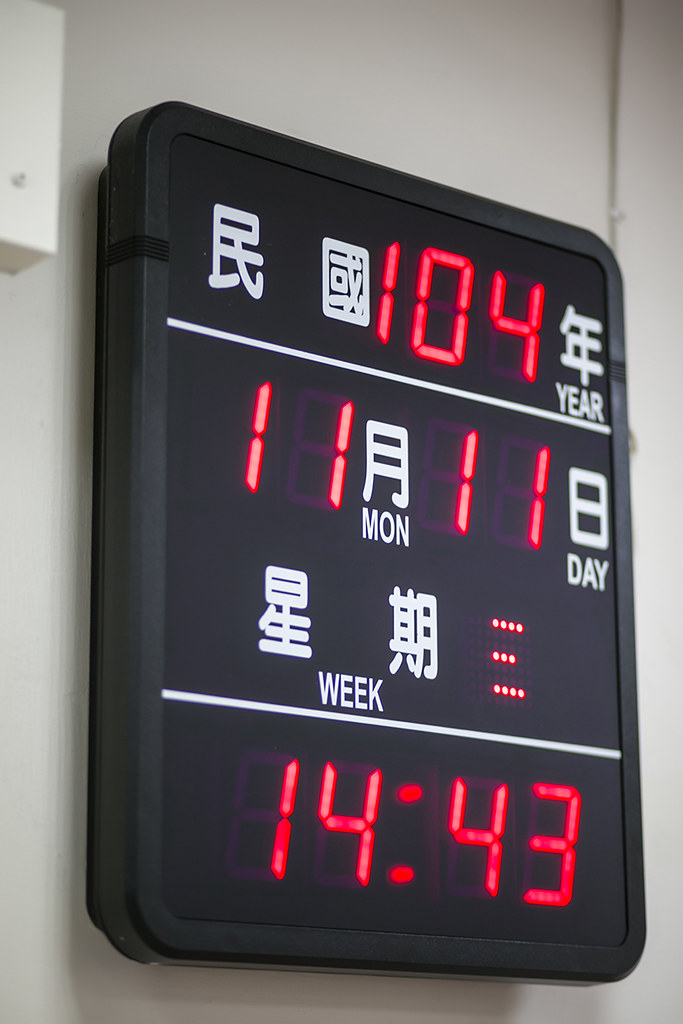This image features a black square electronic scoreboard with white foreign characters dividing it into three distinct sections. The top section prominently displays the digital number "104" in red. Directly below, the middle section shows the numbers "11" and "11" in white. The bottom section of the scoreboard displays a digital time reading "14:43" in white. The entire board maintains a sleek and uniform black aesthetic with a minimalistic design, emphasizing the illuminated numbers and characters against the dark background.